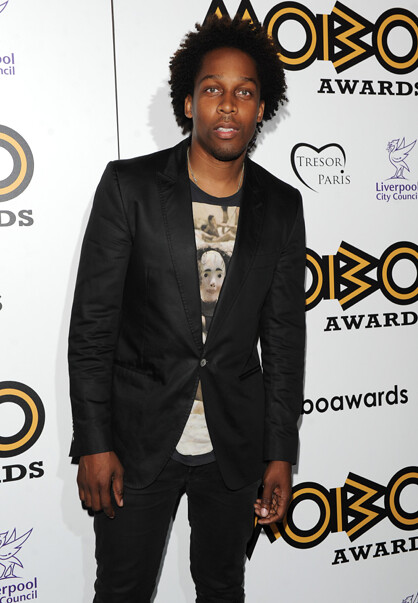The photograph captures an African-American man standing in front of a series of white billboards typically seen at red carpet events, specifically for the Mobo Awards. The primary logo on the billboards reads "Mobo" in yellow with a black outline, and "Awards" below it in smaller black text, repeated multiple times in the background. Additionally, there are other logos, including one from Tresor Paris, featuring a black heart with the text "Tresor Paris" underneath, and another from the Liverpool City Council, which shows a purple bird profile with flapping wings.

The young man at the center of the image is wearing a black blazer, which is buttoned up, concealing most of the graphic design on his t-shirt, although a white mask design is somewhat visible. He pairs the blazer with black jeans and accessorizes with a plain silver necklace. His afro hair is styled into small twists or braids. He stands alone, looking directly at the camera, with no glasses or other jewelry visible. The overall scene conveys a formal yet individualized attire, juxtaposed against the professional backdrop of the award ceremony signage.